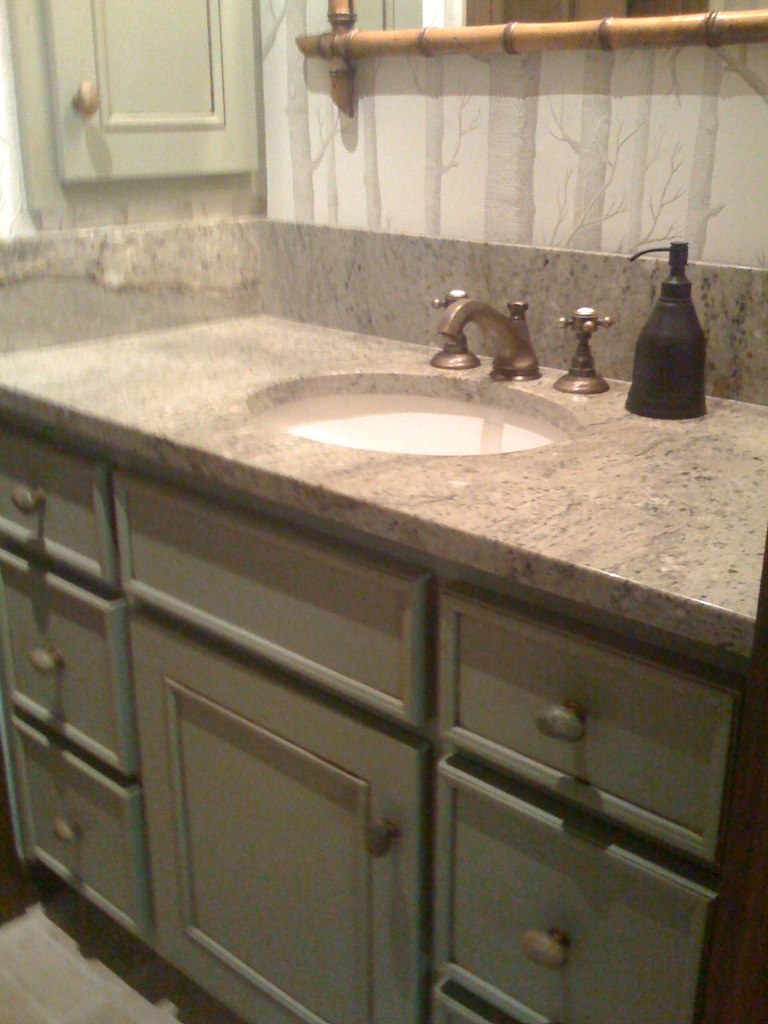The image portrays a somewhat out-of-focus photo of a bathroom vanity featuring a refined and classic design. The vanity boasts a polished granite countertop with an elegant undermount oval sink in a cream or white color. The sophisticated widespread faucet, consisting of separate holes for the left handle, the spout, and the right handle, is designed in an antique style with cross handles and porcelain knobs, likely in a satin nickel finish. The backsplash and left side splash also feature matching granite.

Adorning the countertop is an oil-rubbed bronze pump bottle, presumably for liquid soap, adding a touch of modern contrast. The vanity cabinet appears to be painted in a muted sage green or possibly a gray hue, creating a soft, subtle aesthetic. The cabinet features a central door, providing essential storage, with a false drawer front above to accommodate plumbing.

Flanking the central door are two symmetrical stacks of three drawers, each with an oval pull knob, offering both functionality and streamlined design. There is a hint of a wall-mounted cabinet door above the countertop on the left side, seemingly matching the vanity, although it could potentially be a reflection in a mirror.

The area above the countertop is adorned with wallpaper featuring a serene design of gray tree trunks on a white background. Just visible is the bottom of what is likely a bamboo-framed mirror, although there is a possibility it is a bamboo look towel bar. This coherent mixture of elements creates a serene and timeless bathroom setting.